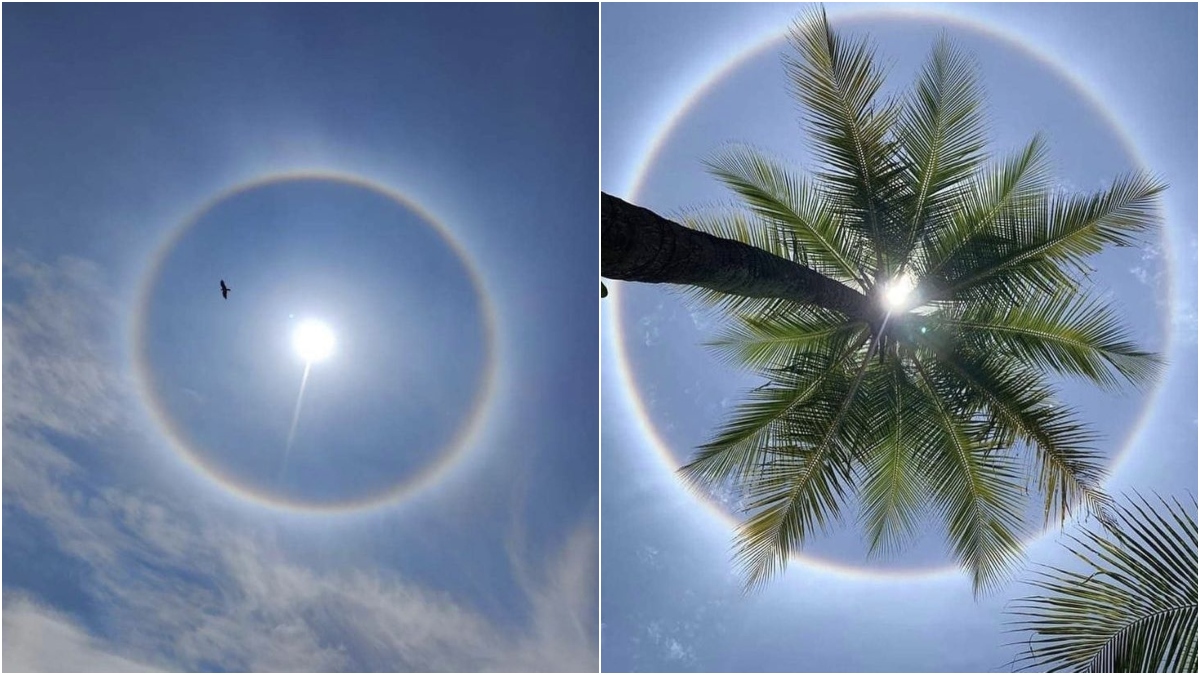The image consists of two side-by-side photographs, both capturing the sun with rainbow-colored halos around it. The left photograph shows a bright white dot at the center surrounded by a colorful halo. Amidst the deep blue sky, there are scattered white clouds and a small black bird flying towards the left. The photograph on the right features a similar sun with a rainbow halo, but includes an upward view of a palm tree. The palm tree's trunk extends halfway down the frame while its fronds stretch out, with light shining through them. The sky in this picture is also blue with some light, wispy clouds. The palm fronds and the surrounding sky create a striking contrast with the circular, colorful halo. The images together emphasize the beauty of the interplay between natural light and the atmospheric phenomena.